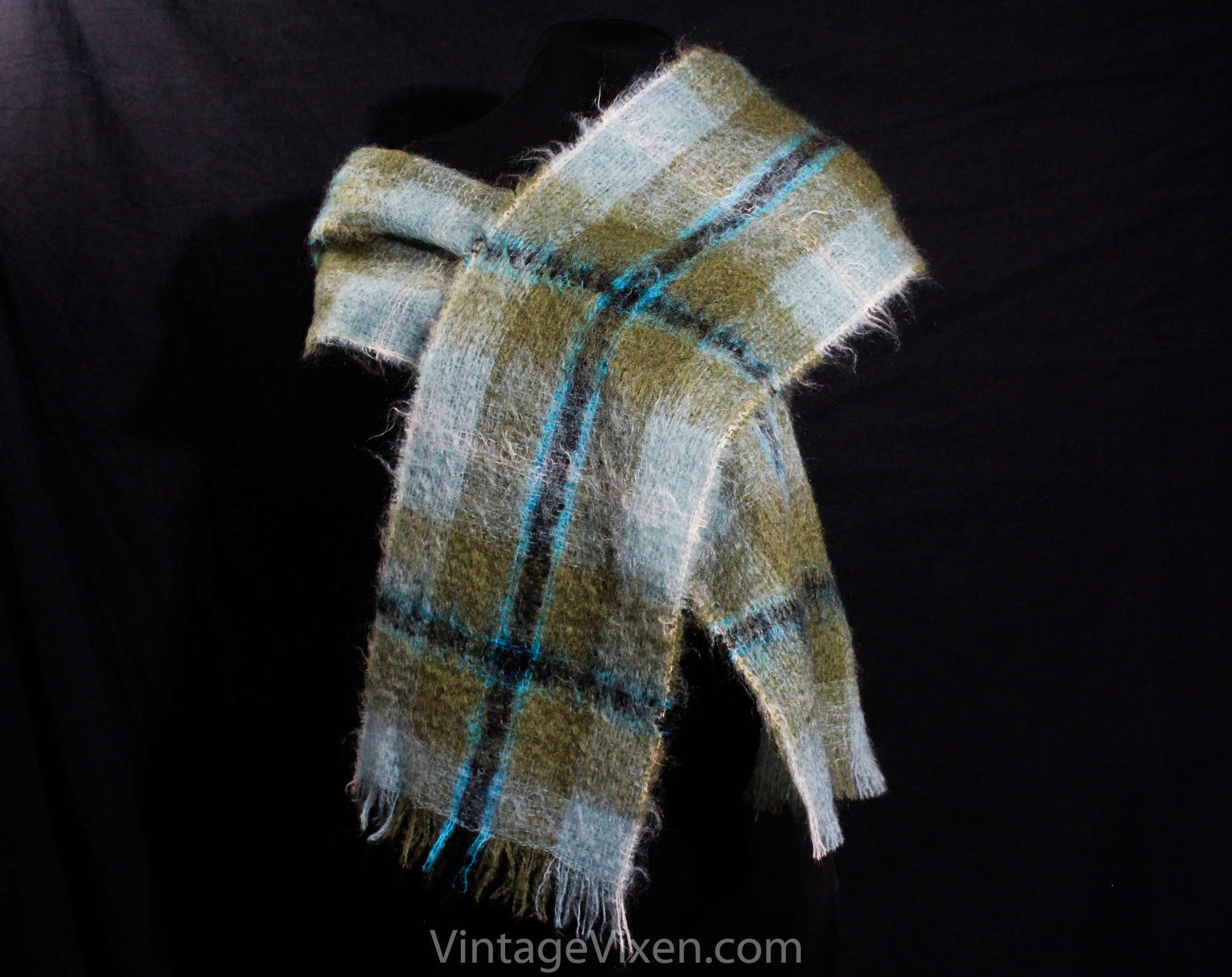The image features a worn, vintage scarf laid atop a black, cloth background. The scarf displays a distinctive checkerboard pattern comprised of white, brown, and black squares. Central to the design is a black stripe running through it, flanked by thin, light blue lines on either side. The checkerboard pattern is further accented by wider brown stripes that add depth to the scarf's intricate weave. The scarf appears to be made of a fuzzy, wool-like material with frayed edges and noticeable tassels at the ends, adding to its vintage charm. At the bottom of the image, white text reads "vintagevixen.com," emphasizing its retro appeal. The scarf's overall appearance suggests it may have been intentionally designed to look old and used, with its frayed look enhancing its nostalgic vibe.